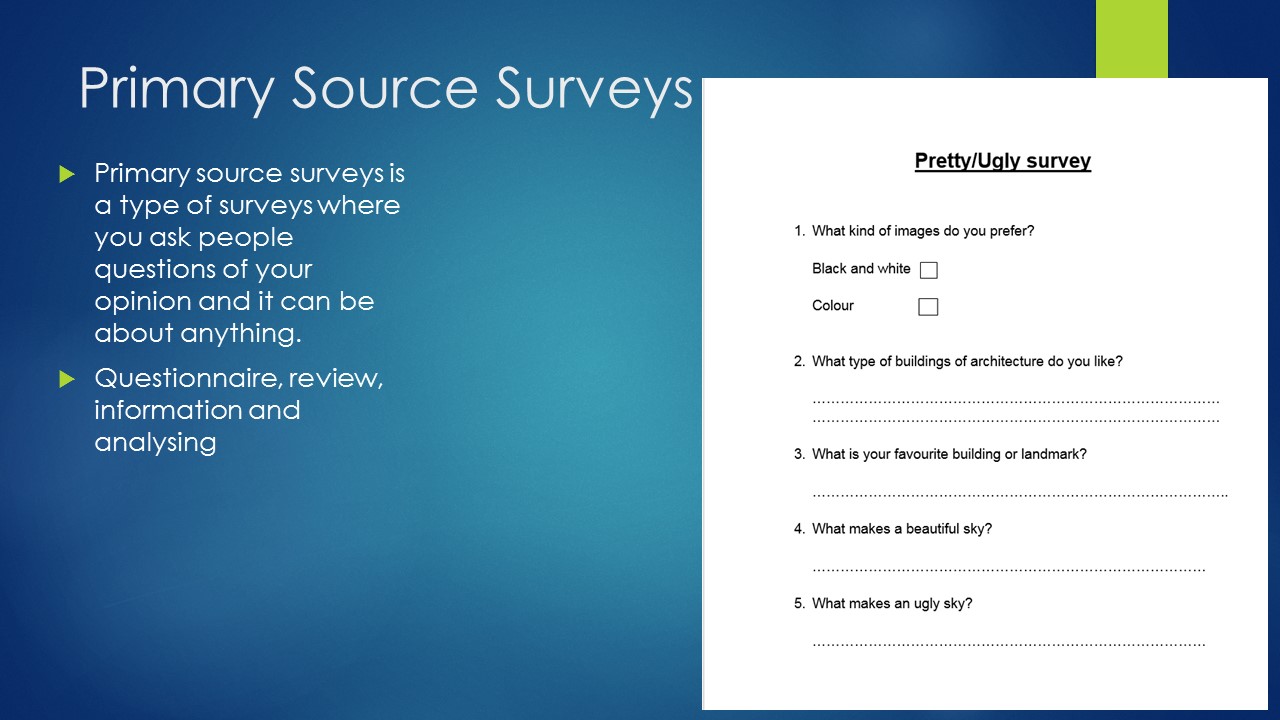The image is a horizontal, rectangular computer graphic, possibly a PowerPoint slide, featuring a survey form against a blue background. In the upper left corner, white text reads "Primary Source Surveys." Beneath this, smaller white text explains that primary source surveys involve asking people questions about their opinions, which can cover any topic. Additionally, it lists "Questionnaire, review, information, and analyzing" with green triangle bullet points. 

On the right side of the image, there's a white vertical section bordered by a light green stripe, resembling a vertical banner. This section contains a form titled "Pretty/Ugly Survey" in black text. The survey consists of five numbered sections: 
1. "What kind of images do you prefer?" with checkboxes for "Black and white" and "Color."
2. "What type of buildings or architecture do you like?" followed by two blank lines for responses.
3. "What is your favorite building or landmark?" with one blank line for an answer.
4. "What makes a beautiful sky?" accompanied by one blank line.
5. "What makes an ugly sky?" again with one blank line for a response.